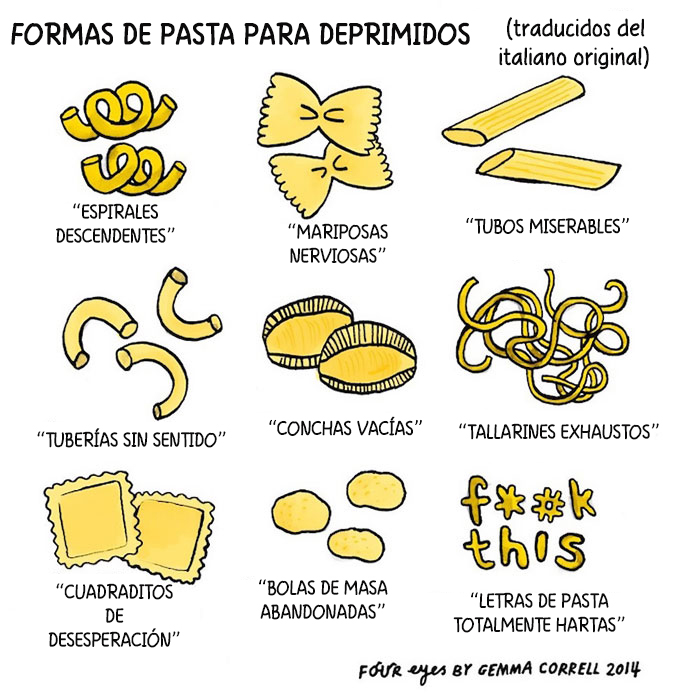The image, titled "Formas de pasta para deprimidos" (Types of Pasta for Depressed People), humorously depicts nine different types of pasta, each with a whimsical, melancholic twist in their Spanish names. The entire illustration is set against an all-white background, with black text. Below the title, a subtitle states “Traducidos del Italiano original,” suggesting a translation from original Italian names. Arranged in a three-by-three grid, the pasta types and their translations are as follows: 

1. "Espirales descendentes" (Downward Spirals) depicted as spiral pasta.
2. "Mariposas nerviosas" (Nervous Butterflies) illustrated with butterfly-shaped pasta.
3. "Tubos miserables" (Miserable Tubes), which look like penne.
4. "Fideos sin sentido" (Pointless Noodles), showing regular spaghetti.
5. "Conchas vacías" (Empty Shells), represented by shell pasta.
6. "Tallarines exhaustos" (Exhausted Tagliatelle), shown as thick, flat noodles.
7. "Raviolis abandonados" (Abandoned Ravioli), illustrated as ravioli pasta.
8. "Bolas de masa desechadas" (Discarded Dough Balls), depicted as small pasta balls.
9. "Letras de pasta completamente hartas" (Totally Fed Up Pasta Letters), featuring alphabet pasta.

The illustration ends with the somewhat aggressive text, "Fuck this," emphasizing the bleak humor. At the bottom, it is credited to "Four Eyes by Gemma Correll, 2014."